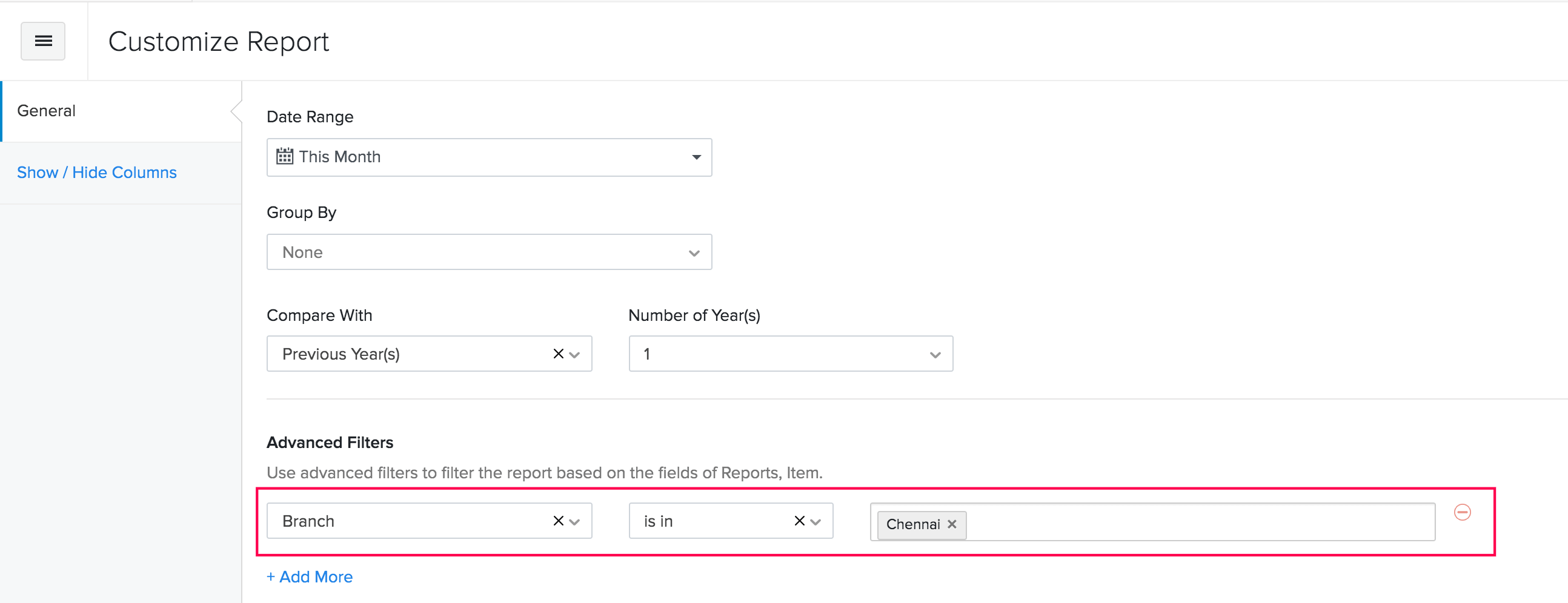The image displays the top section of a user interface for customizing reports. Positioned towards the left is the header "Customize Report," written in black text. Directly left of this heading is a square containing three horizontal black lines, likely representing a menu icon. A vertical line separates the menu icon from the "Customize Report" text, although they are adjacent at the very top of the interface.

Beneath the menu icon, two headings are visible: "General" at the top in black text and directly below it, "Show/Hide Columns" highlighted in blue. 

Adjacent to these on the right, the interface includes a set of dropdown menus and options. "Date Range" is followed by the option "This Month" within a box. Below this, "Group By" is listed with "None" selected. The next option, "Compare With," offers "Previous Years" in a box. Further right, "Number of Years" has the value "1" displayed in a box. 

A horizontal line separates these sections from the next segment titled "Advanced Filters", which is in black text while the surrounding text appears in gray. A description underneath reads, "Use Advanced Filters to filter the report based on the field of reports item." This section is enclosed in a red outline, and within it, there is a box containing the options "Branch," "Is In," and "Channel."